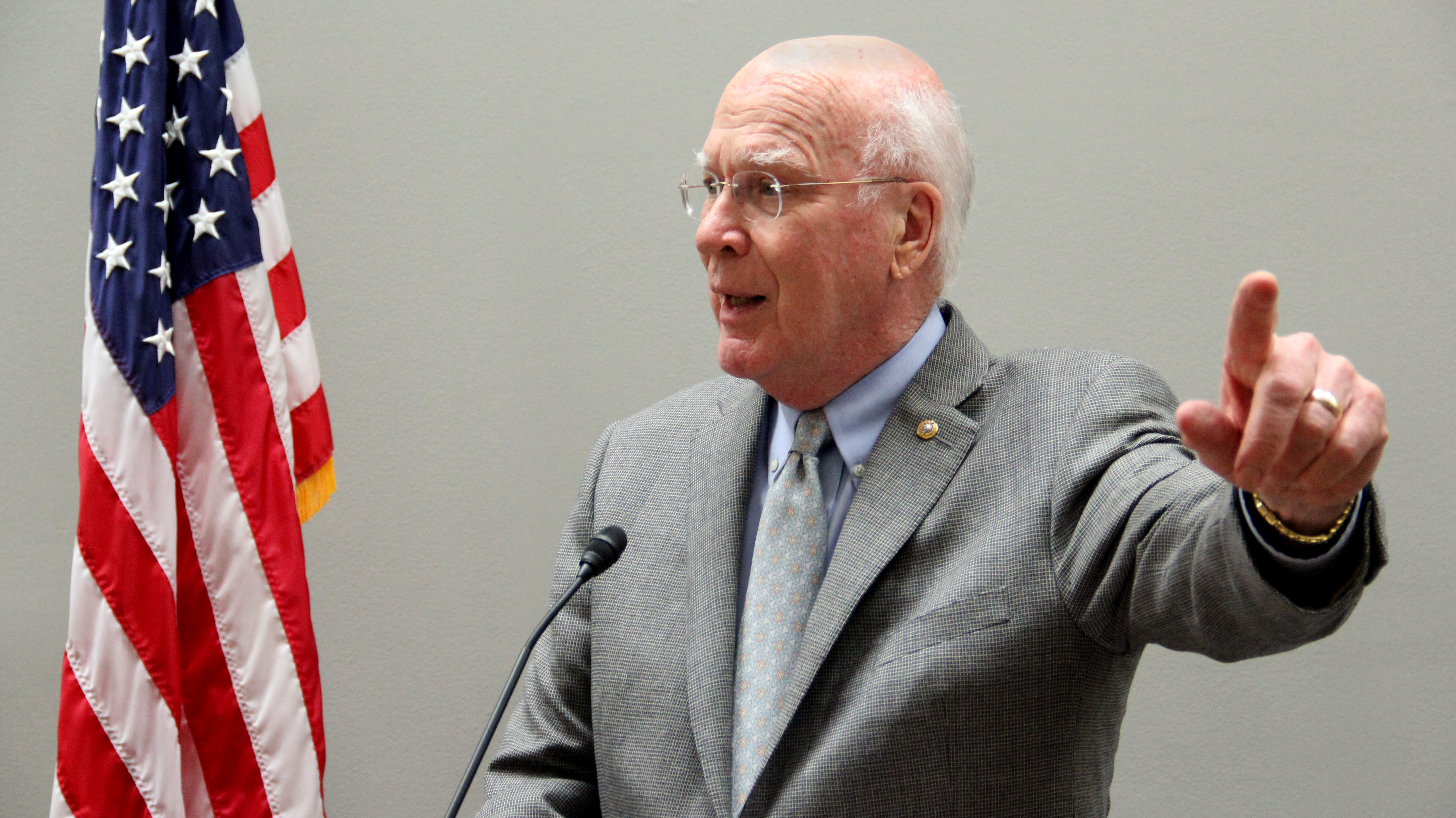The image features Senator Patrick Leahy of the United States, captured mid-speech. He is wearing a light gray suit with a matching tie and a light blue collared shirt underneath. A distinctive golden pin adorns his jacket, and on his left wrist, he wears a golden watch or bracelet. Senator Leahy, an older man with white hair around the back of his head and bald on top, is seen pointing with his left hand, which also bears a wedding ring on the middle finger. He is wearing glasses, and his mouth is open as if he is speaking. In front of him is a thin black microphone, positioned slightly to his left, and an American flag drapes downward in the background. The surroundings and details suggest an indoor setting.